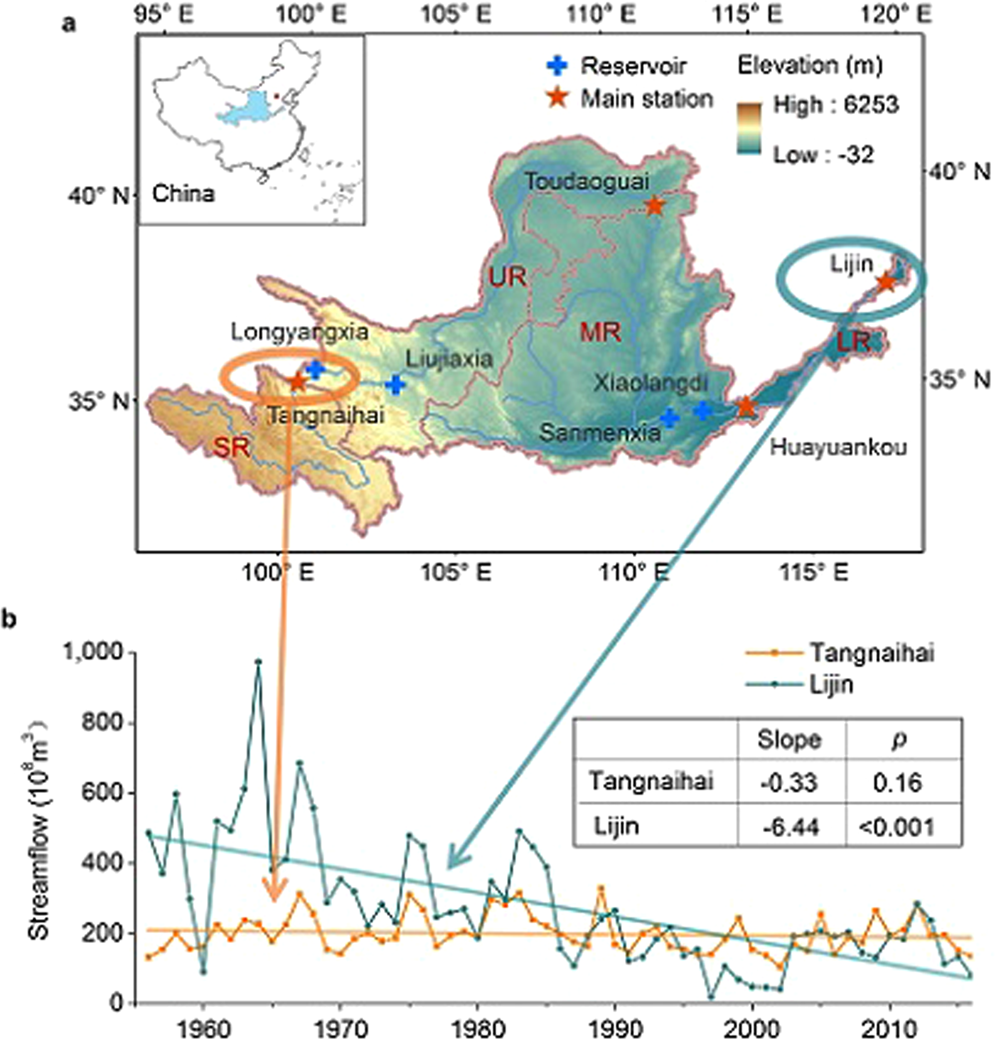The image features a dual-infographic presentation overlaid on a map that specifically highlights a region within China. In the upper section, a physical map showcases the topographical variances of the land, represented through a color gradient ranging from green for low elevations to brown for higher altitude areas. A key located at the top of the map deciphers various symbols: a blue plus sign indicates reservoirs, while a red star marks the main station. 

The map primarily focuses on a specific part of China, demarcated in blue in the top-left corner to distinguish the highlighted region from the rest. 

The lower section supplements the map with a graph featuring stream flow data over time. The horizontal axis signifies the years, while the vertical axis measures stream flow in a grayscale format. This graph contains plotted data from two distinct locations within the highlighted region, illustrating temporal variations in stream flow.

Essentially, this comprehensive visual merges geographical and hydrological information, providing insights into both the terrain and the stream flow trends of a particular area in China across different years.